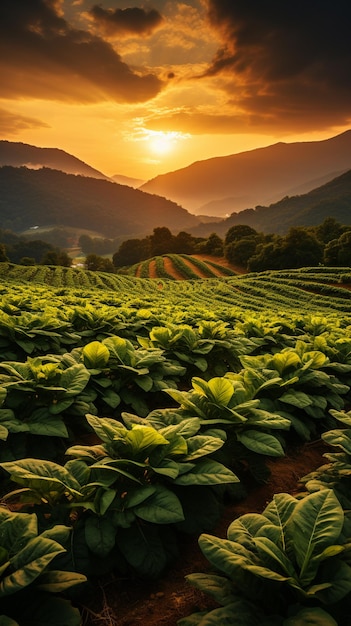The image captures a lush agricultural field filled with rows upon rows of vibrant green leafy crops, possibly resembling spinach or salad greens. The foreground reveals a patch of brown dirt, indicating freshly tilled soil, while the uniform rows of crops stretch seamlessly towards the horizon. In the background, the terrain transitions into hilly areas adorned with large, verdant trees that exhibit a full, healthy appearance. Beyond these hills, the silhouette of more distant, dark hills contrasts with the dramatic sky above. Heavy clouds, tinged with the golden hues of the setting sun, create a striking atmosphere, as the sun dips below the horizon, bathing the scene in exquisite, warm light. The intricate interplay of light and shadow, along with the meticulous arrangement of the plants and natural elements, lends a serene and picturesque quality to the landscape.